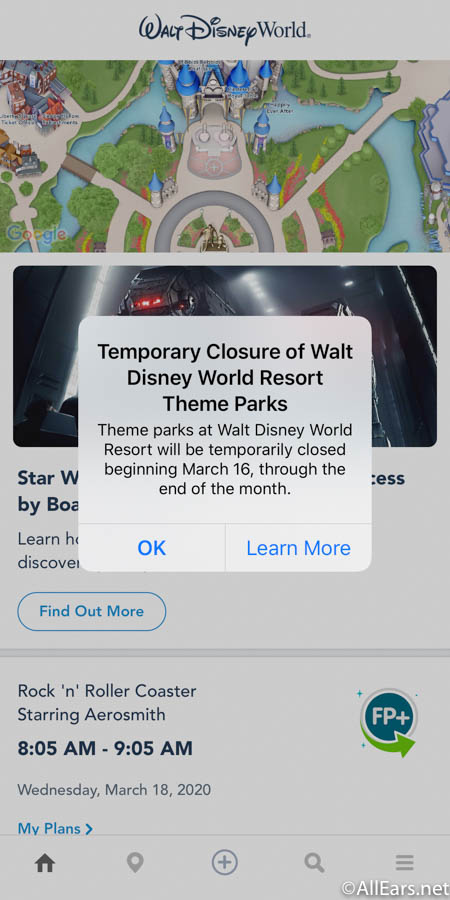This is a detailed screenshot of a mobile or tablet-formatted website interface displaying information about the temporary closure of Walt Disney World Resort theme parks. The background has a greyish hue and features various images and texts. Prominently in the center is a slightly translucent, white pop-up window that partially obscures the background, which includes a black and red image, likely related to Star Wars. The pop-up window announces the temporary closure of Walt Disney World Resort theme parks, stating, "Theme parks at Walt Disney World Resort will be temporarily closed beginning March 16 through the end of the month." Beneath this announcement are two clickable buttons: "OK" on the left and "Learn More" in a blue box on the right. 

Behind the pop-up, at the very top center, the Walt Disney World logo is visible. The background image appears to be a stylized, almost cartoon-like, bird's-eye view of the theme park, complete with trees, walkways, castles, and a river. Directly below, partially obscured by the pop-up window, is a dark logo featuring a red-eyed robot and text that includes a stylized "Star W" indicating a Star Wars theme. Beneath this logo is a blue-edged button labeled "Find Out More."

Further down, written in black text, is information about a specific ride: "Rock 'n' Roller Coaster Starring Aerosmith: 8:05 AM to 9:05 AM, Wednesday, March 18, 2020," with "My Plans" highlighted in blue to its right. Nearby, a blue circle labeled "FP+" in white features a curved green arrow underneath it, indicating some sort of interactive feature.

At the very bottom of the screen are phone icons representing Home, Location, Plus, Search, and a Hamburger Menu. In the bottom right-hand corner, partially visible, is a white watermark that appears to read "Copyright AIBR" in white text.